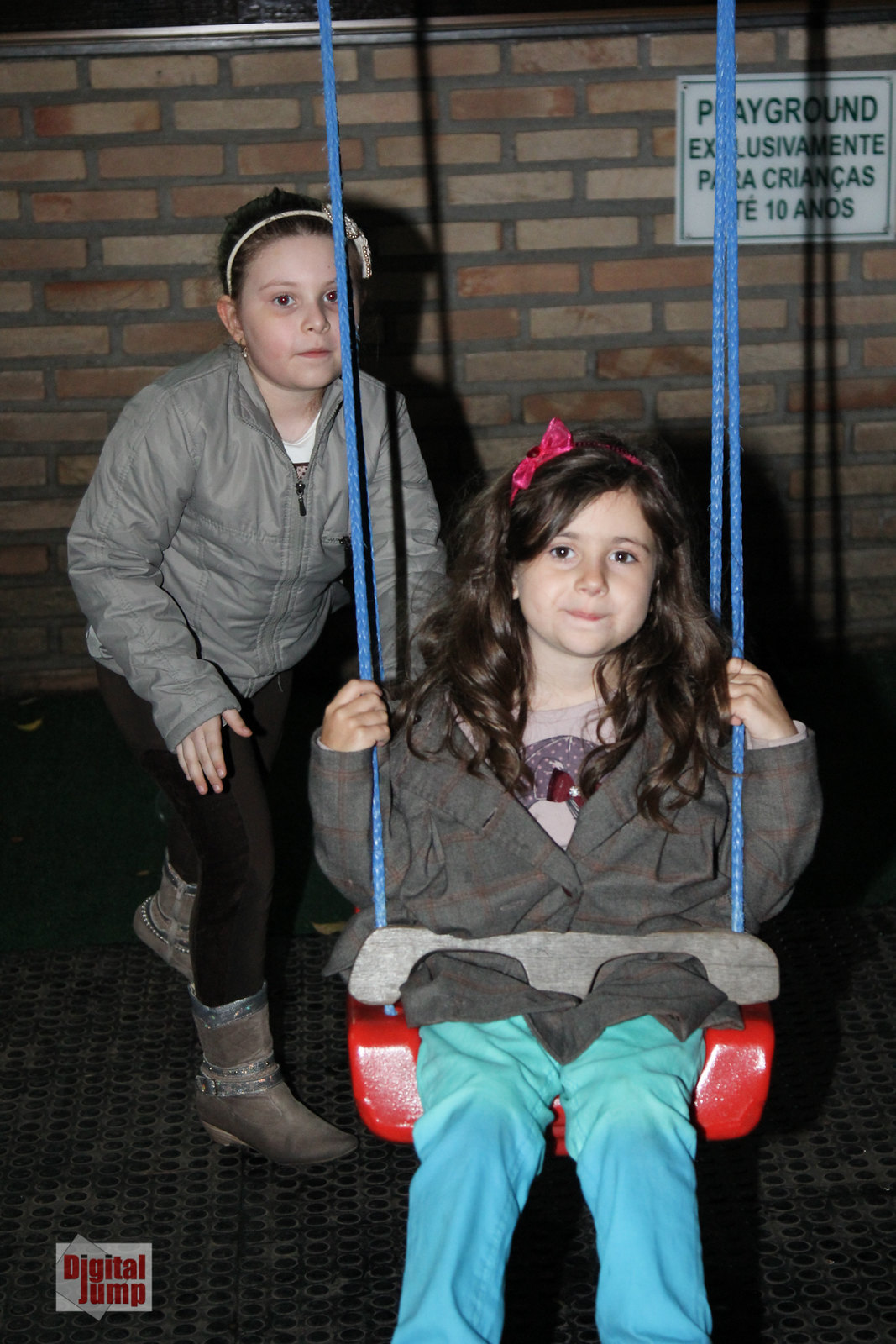The image depicts two young girls in front of a brick wall with a mix of gray and orange bricks and dark gray mortar. In the foreground, a girl with long dark brown hair, parted on the right and falling just below her shoulders, is sitting on a red swing with blue ropes. She is wearing a gray jacket and light blue pants, and she has a soft smile framed by a red bow in her hair. Behind her stands another young girl, who appears to be her sister, wearing a light gray jacket, black pants, and gray boots. She has her hair tied back tightly with a white hairband, which reveals her ears, and she seems to be gently pushing the girl in the swing with her one visible hand. The ground beneath them is a dark gray rubber mat with black spots. In the upper right corner of the image, there is a white plaque on the wall featuring black text in a foreign language, possibly Spanish, that includes the word "Playground" and phrases like "Exclusivamente Para Crianacas," along with some obscured words. In the bottom left corner, a white box with red text reads "Digital Jump." The overall setting hints at a playground, potentially located indoors or captured at night, given the shadowy ambiance.